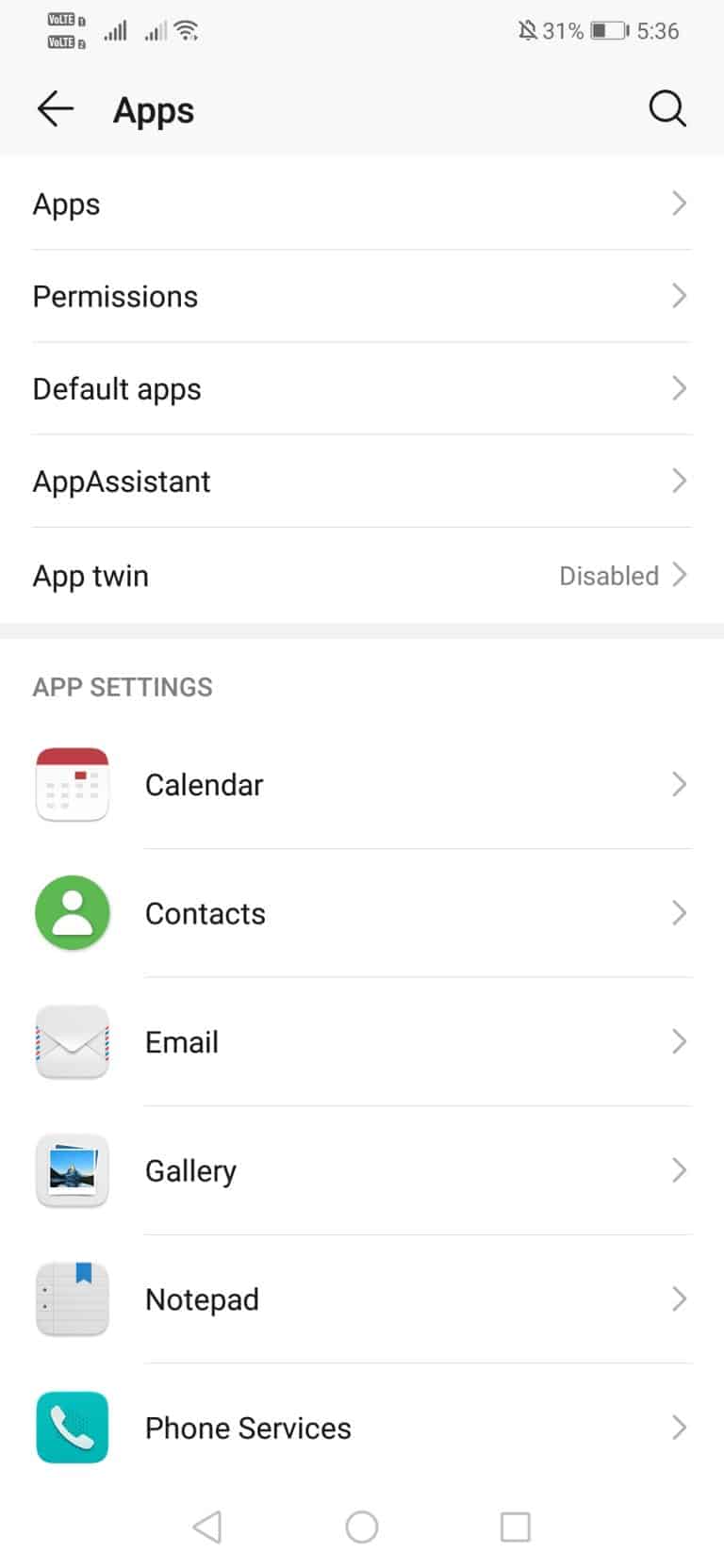The image showcases a screenshot of an Android phone's settings menu, specifically within the "Apps" section. At the top of the screen, we see the title "Apps" alongside a back arrow, helping to identify the navigational context of this page. There is a search icon (magnifying glass) to the right for easy navigation within the section. 

The status bar displays the time "5:36" along with a battery indicator showing 31% remaining battery life. It also indicates that notifications are turned off, as evidenced by the crossed-out notification bell icon. Connectivity icons reveal that the phone is connected to Wi-Fi and is using an LTE network.

The main part of the screen is divided into several sub-sections, starting with "Apps" and "Permissions," each accompanied by navigational buttons leading to further details. Next, there are sections labeled "Default Apps," "App Assistant," and "App Twin," with the latter noted as being disabled. 

Below these categories, there is an "App Settings" section that lists specific applications such as Calendar, Contacts, Email, Gallery, Notepad, and Phone Services. Each of these apps is accompanied by distinct, recognizable icons: a calendar for Calendar, a silhouette for Contacts, an envelope for Email, a stack of pictures for Gallery, a notepad for Notepad, and a phone for Phone Services.

The user interface has a minimalist design with a white background, black text, and various small, colorful icons representing each app. This clean layout ensures easy readability and straightforward navigation for the user.